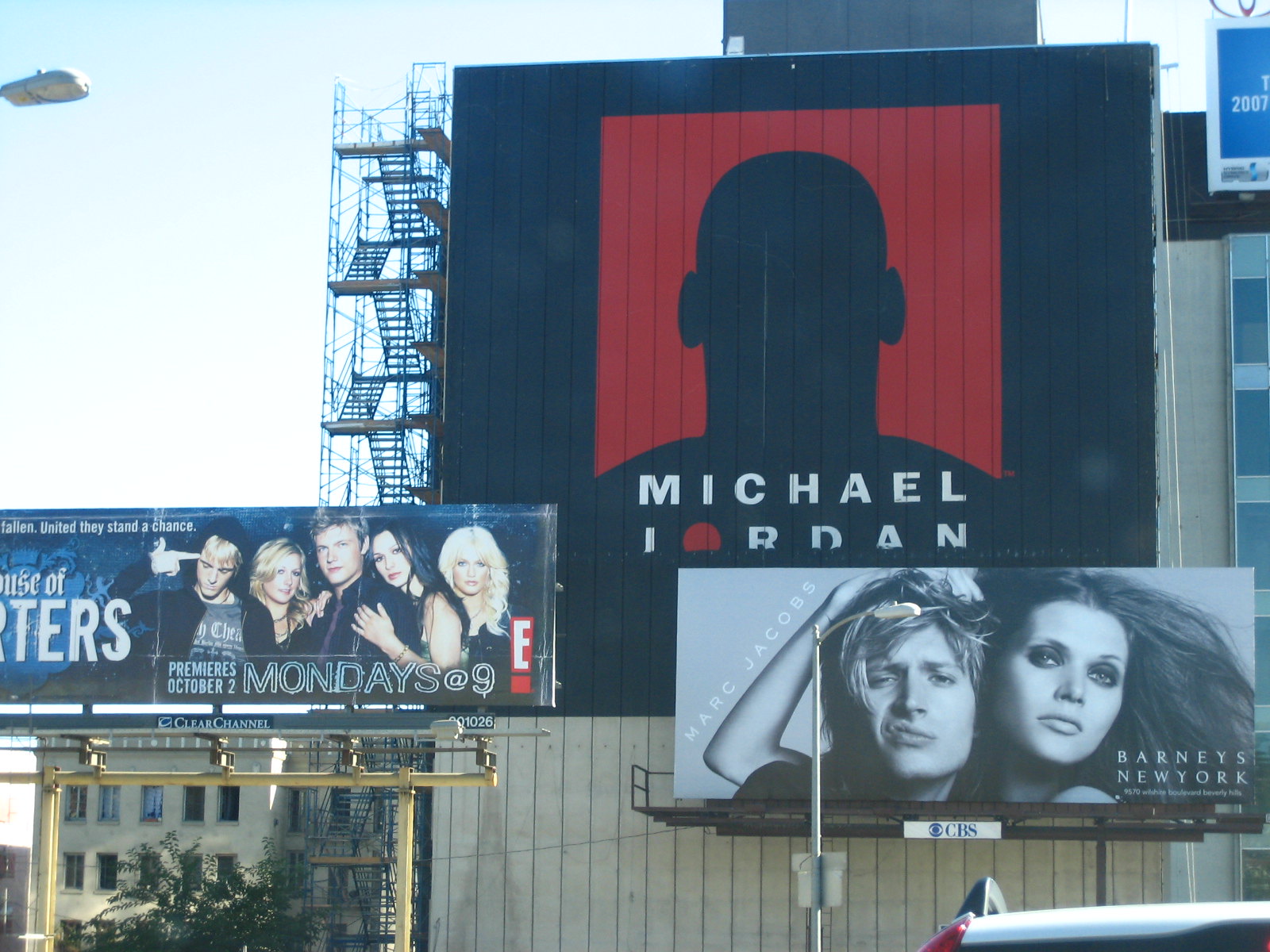The image showcases three distinct billboards prominently displayed against an urban backdrop. The highest billboard features an iconic silhouette of basketball legend Michael Jordan. The background is primarily black, with a striking red square on which the dark, silhouetted figure of Michael Jordan is superimposed, exuding a sense of mystery and reverence.

Below this, another billboard advertises a television show with the text "Premieres October 2nd, Mondays at 9." The display includes five individuals—two men and three women—lined up to promote the show, suggesting an ensemble cast.

The third billboard promotes Barneys New York, showcasing a stylish image of a Caucasian male and female, possibly models, epitomizing sophistication and elegance. Below this billboard, there's a small logo of CBS, accompanied by the CBS eye symbol, indicating collaboration or sponsorship by the television network.